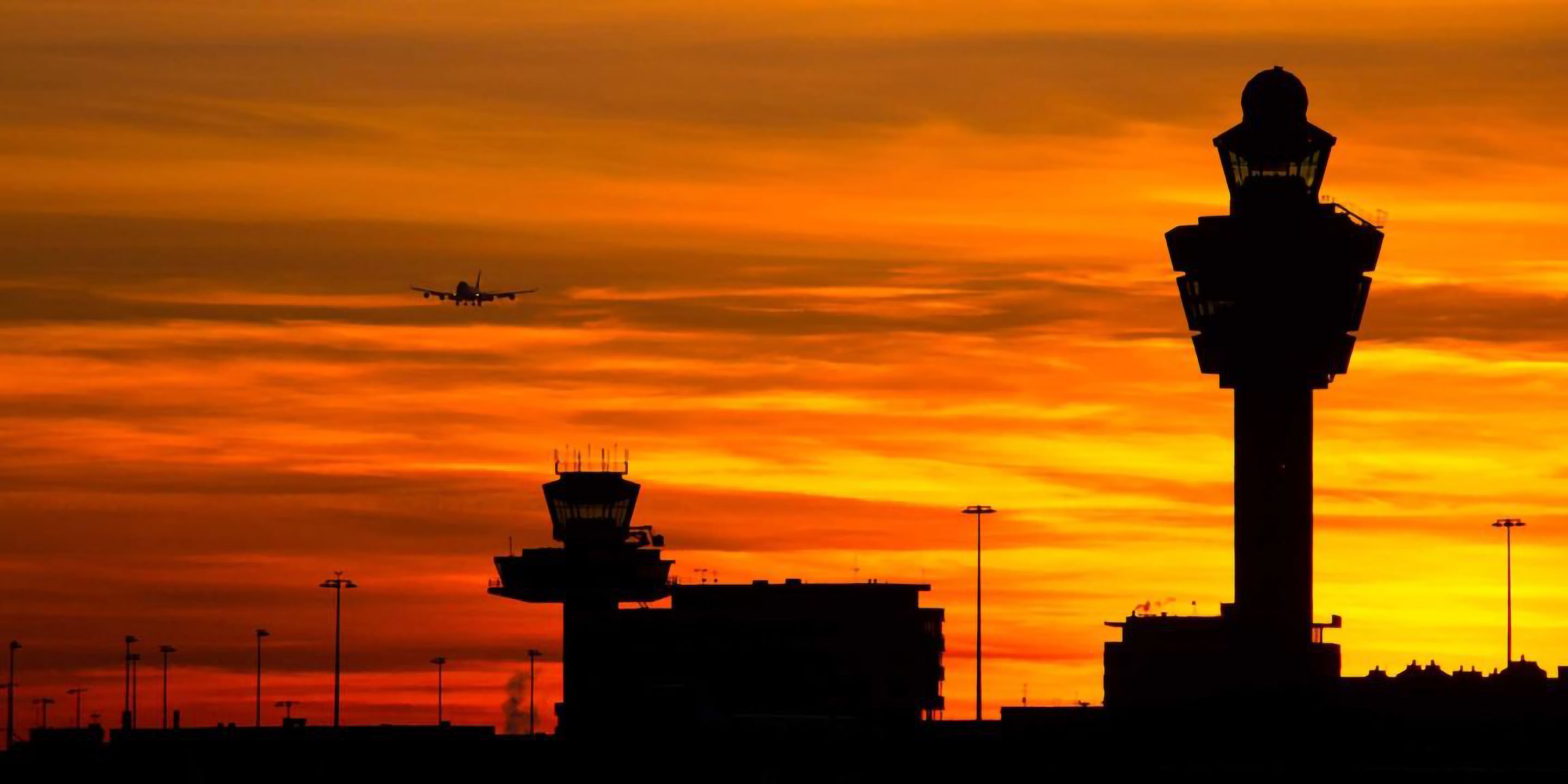This photograph captures a vivid and realistic scene of an airport at sunset, oriented horizontally in a rectangular format. The sky is a mesmerizing blend of reds, oranges, yellows, and browns, illuminated by the low sun, casting a golden glow across the horizon. Scattered clouds enhance the striking colors, reflecting the warm hues. A large airplane, silhouetted against the vibrant sky, appears to be flying towards the camera.

In the darkened foreground is the silhouette of an airport complex. Dominating the scene are two control towers: one tall and prominent to the right, with a narrow top and wider base, and another, shorter or more distant, positioned towards the center. These towers, shrouded in shadows due to the backlighting, stand as sentinels over the scene.

Flanking the landscape on the left are several high light poles, likely illuminating the tarmac or parking lots. Also visible are other smaller structures, including squared-off buildings and what might be speaker or light posts with distinctive features suggesting multifunctional use, though details are obscured in silhouette.

The overall impression is one of serene, twilight beauty, capturing both the utility of an airport and the natural splendor of a sunset.